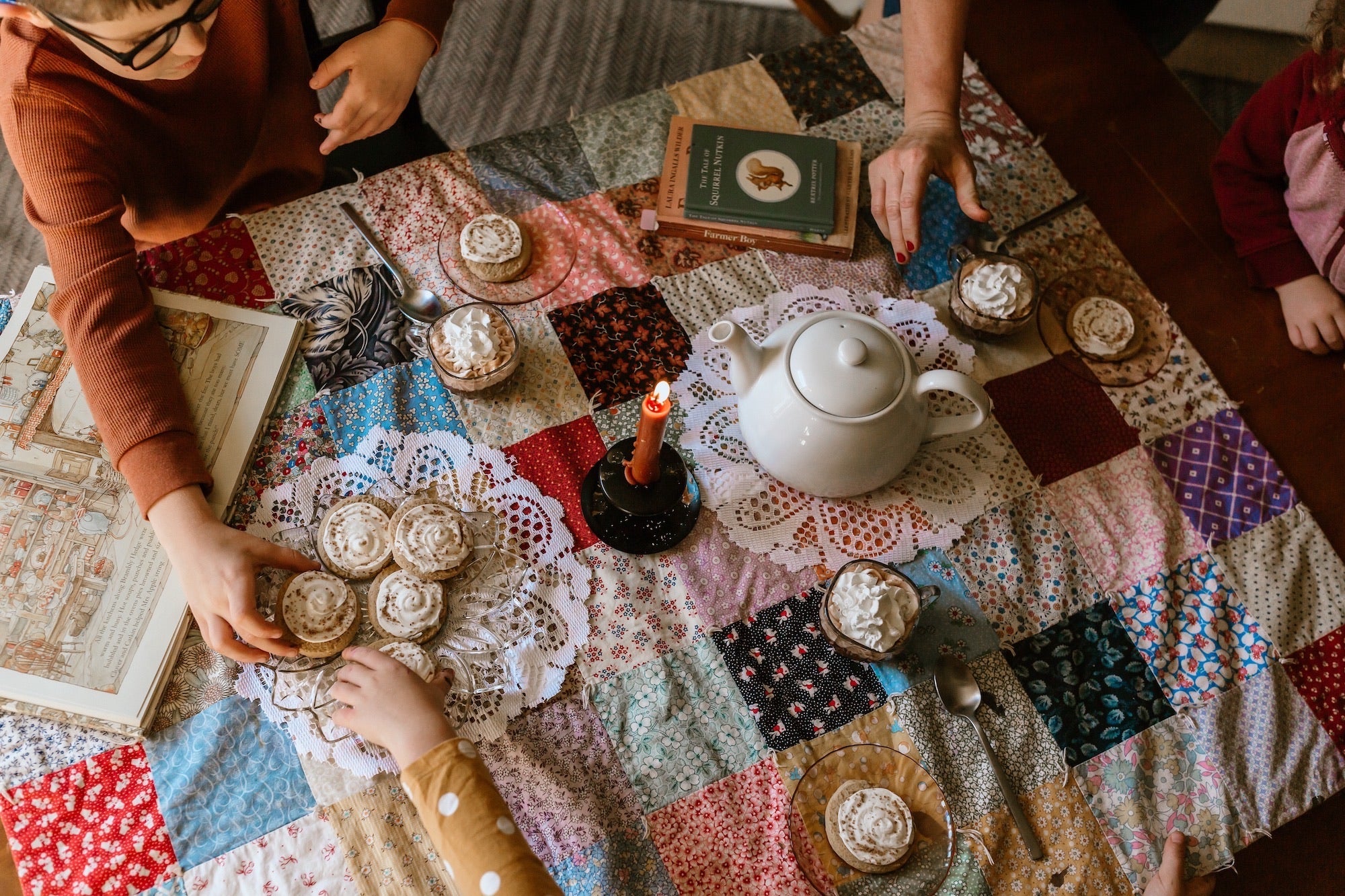This overhead image captures a vibrant, cozy gathering around a table adorned with a colorful, patterned patchwork quilt. The table is a delightful mosaic of colors, featuring predominantly brown, white, red, purple, light blue, light green, and black hues. At the center, an orange candle on a black base adds a warm glow to the scene. Surrounding this focal point are various items, including a green book atop a light brown one and numerous small plates with frosted cookies and pastries.

Three people are partially visible in the image. One woman, identifiable by her short hair, black glasses, and long-sleeved light brown shirt, is in the process of picking up a cookie. To the top right, another individual with a long-sleeved purple shirt extends a right hand towards the assortment of desserts. At the top left, a young boy wearing glasses reaches out for a cookie with frosting.

Amidst the intricate embroidery of the quilt are doilies placed below a beautiful glass petaled plate with desserts and a white teapot, enhancing the table's inviting charm. Another right hand reaches from the bottom left, wrapped in a long-sleeved orange polka-dotted shirt, possibly belonging to another child. The scene is a rich tapestry of community, comfort, and color, centered around a shared moment of enjoying tea, treats, and each other’s company.